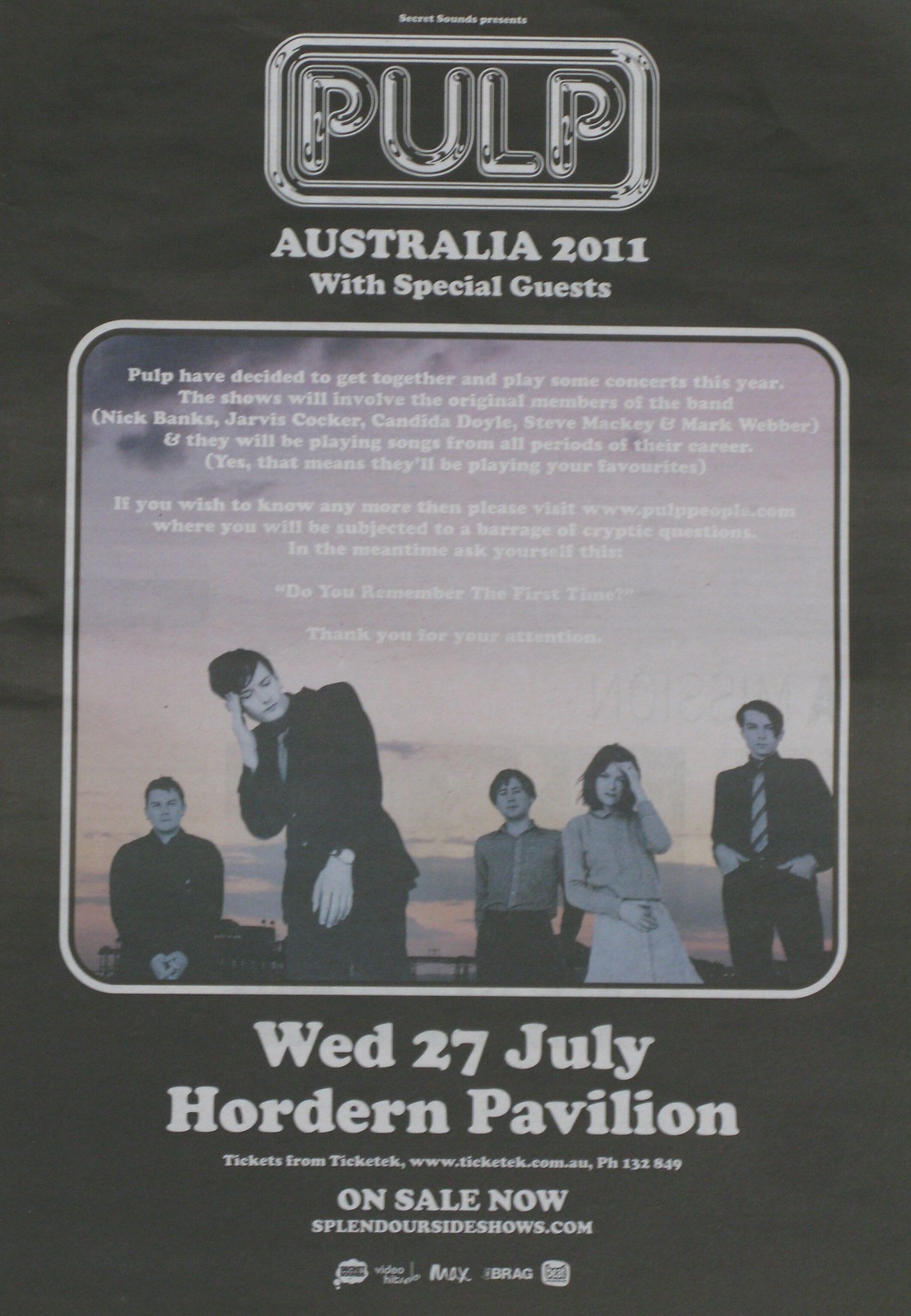This poster, set against a black background with striking white text, advertises a 2011 Pulp concert in Australia. At the top, "Secret Sounds Presents" leads into a stylized, glass-like "PULP" logo inside a rounded rectangle. Beneath it, the poster declares, "Australia 2011 with Special Guests." The central focus is a large photo featuring the five original band members—Nick Banks, Jarvis Cocker, Candida Doyle, Steve Mackey, and Mark Webber—posed against a dusk sky. The photo is mostly black and white, except for the sky, adding a dramatic backdrop. Accompanying text explains that Pulp has reunited for concerts, promising to play favorites from all periods of their career. Additional information and quirky commentary direct readers to visit www.pulppeople.com for more details. The bottom portion of the poster provides specifics about the concert: "Wednesday, 27th July, Hordern Pavilion," with ticket purchase information from Ticket Tech (www.tickettech.com.au, phone 132 849) also noted.